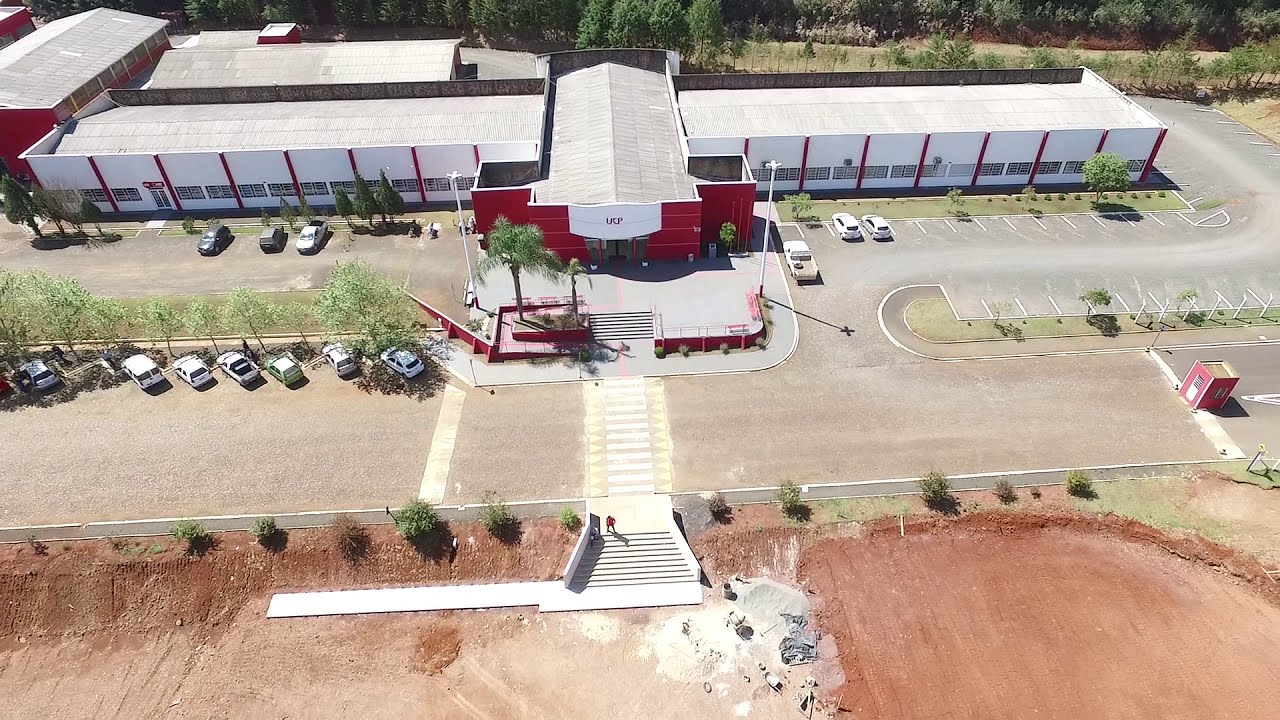This aerial photograph showcases a newly constructed, sprawling commercial or educational complex, potentially a high school or company headquarters. The central focus is a large two to three-story building with a red front and white sides, forming a T-shape with horizontal wings extending from both sides. The building features a flat gray roof with a slight A-frame in the middle and a white awning above the main entrance displaying red "UCP" lettering.

To the left of this primary structure, another red and white vertical building stands adjacent. A well-marked parking lot surrounds the building, complete with fresh stripes and several parked cars. The parking area extends and wraps around to the right side.

In the middle of the image, a crosswalk leads to a set of white concrete stairs, where a person is seen ascending. The stairs connect to the main building, positioned between the asphalt street at the bottom and the central complex. Beyond the main structures, there is a dirt field, presumably for a track or football field, emphasizing the newness of the development. Additional surrounding buildings further frame the scene, enhancing the complexity of the site layout.